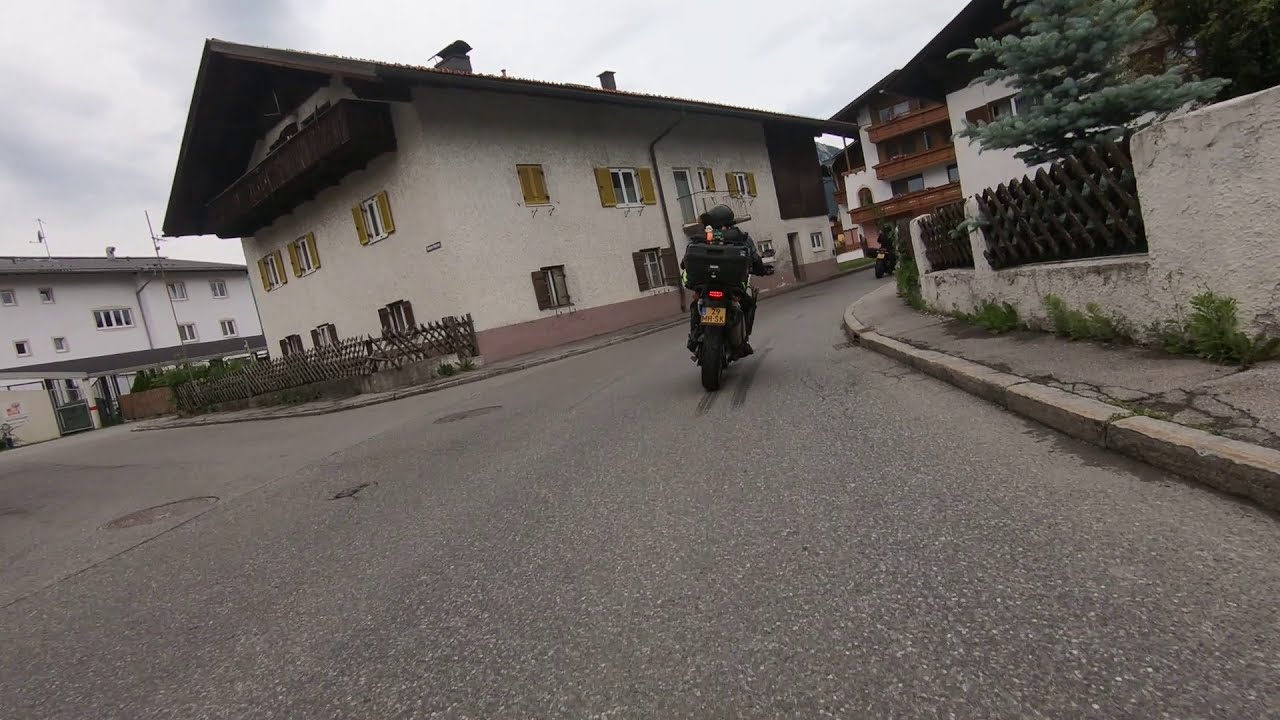The image showcases a city street scene where a black motorcycle, which has a yellow license plate, is the central focus. The motorcycle, ridden by a driver in a black helmet and all-black attire, is curving to the right and moving towards the top right corner of the image. Notably, there is another motorcycle further ahead, about to disappear from view. Both riders are dressed in black. The street itself has a cracked sidewalk on the right side and is lined by buildings on both sides. 

To the left, there is a distinctive off-white, two-story building with green shutters, a triangular dark brown roof, and a prominent plant hanger. This building also features a spiked fence around its front left side. Further back on the left, another white building is visible, but details are obscured. On the right, the road is bordered by a stone fence with concrete pillars, leading to another building, though it’s not clearly visible. The sky peeks through in parts of the background, adding to the urban landscape. The photograph is slightly angled, adding a dynamic perspective to the city environment.